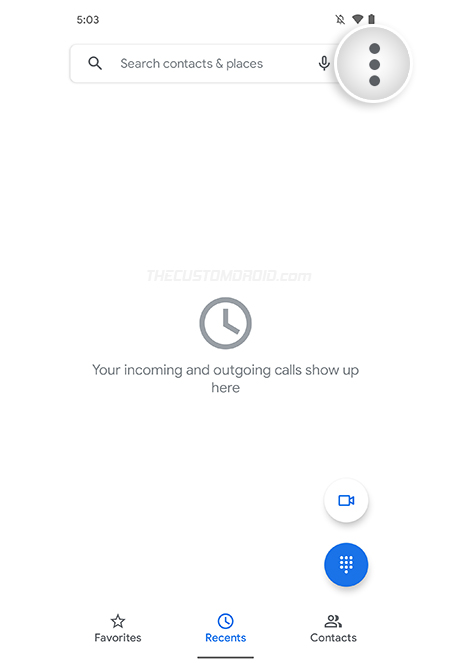A detailed caption for the described image could be:

"This image depicts a minimalistic and primarily white phone screen interface, specifically the call log screen. The background is predominantly white with grey text annotations and various simple icons. At the top of the screen, the status bar displays the current time, battery level, and signal strength indicators. Directly below, a search bar labeled 'Search contacts and places' is present, accompanied by a three-dot menu icon that suggests additional options can be accessed by tapping it. 

Central to the image is a prominently larger club icon with accompanying text stating, 'Your incoming and outgoing calls show up here,' indicating that this section is meant to display call logs. However, the screen is currently empty, signifying that no calls have been made or received yet.

Near the bottom of the screen, several navigation icons are displayed. From left to right, these include: a star icon representing 'Favorites,' a clock icon indicating 'Recent' calls, and a contacts icon symbolizing two simplified figures to denote the 'Contacts' section. Additionally, a small camera icon is also visible, presumably for access to the camera feature.

Overall, the interface is straightforward and uncluttered, emphasizing simplicity and ease of use."